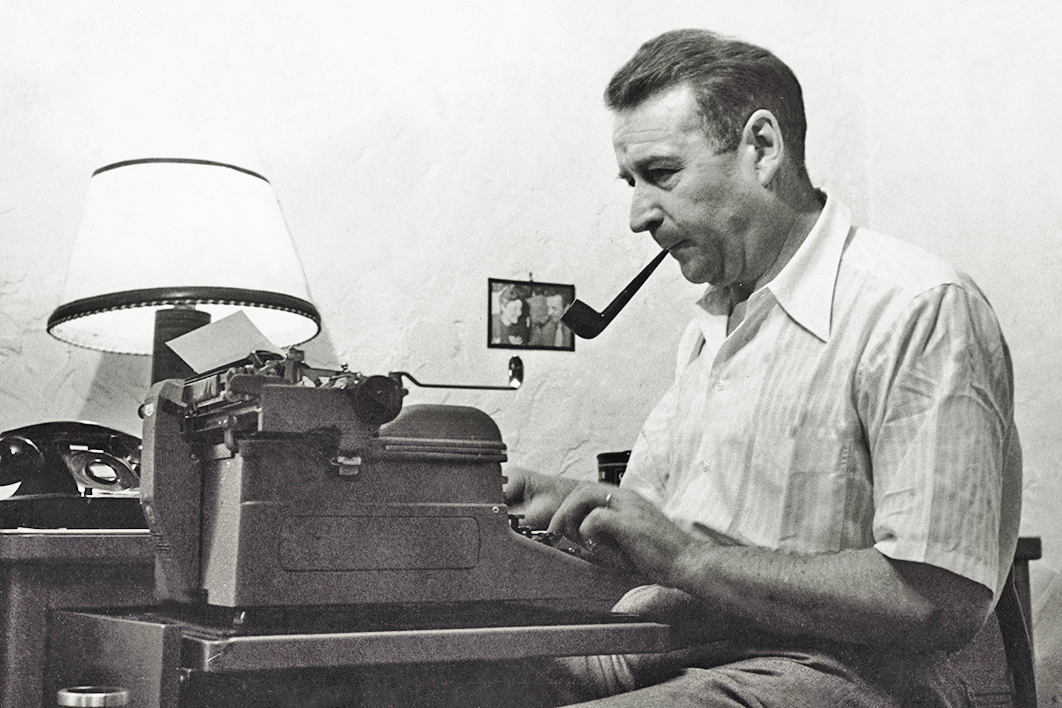In this rectangular black-and-white photo, slightly more long than tall, an older man, likely in his mid-to-late 40s or early 50s, sits on the right side, facing left, and typing on a vintage mechanical typewriter. The man, who has short brown hair and muscular arms, is dressed in a white short-sleeved button-down shirt with some stripes and light-colored pants. He holds a wooden pipe in his mouth, suggesting he is a smoker. His hands appear motion-blurred, indicating he is in the act of typing. The typewriter is positioned on a slide-out drawer of the desk, creating an old-time office scene. Behind him, the desk holds a black rotary phone and a lamp, underlining the period's ambiance. On the wall behind him, which is white, there is a small picture of presumably the same man with a woman, with the man identifiable by the pipe in his mouth. The well-lit room offers a glimpse into the mid-20th century, completing a nostalgic and detailed snapshot of an era gone by.